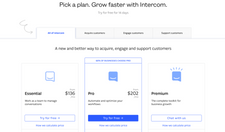The image appears to be a zoomed-in section of a website that details pricing plans for a service, likely Intercom. At the top, small black text reads "Pick a Plan: Grow Faster with Intercom." Below this header, there are four subcategories, though they are small and blurry. Of these, one subcategory is highlighted in blue text, while the others are in black.

Further down, bold black text states, "A new and better way to engage and support customers." Directly beneath this is a square section containing an image of a chat box with a price label of $202. Adjacent to this is a long blue rectangle, which seems to be a clickable button to activate the plan.

On the left side of the image, another section labelled "Essential" includes a square with a smiley face icon and the price $106. Over to the right, another area labeled "Premium" is presented with a blue square containing a smiley face icon and "Premium" in bold black text. Underneath this label, there are two rows of very small black text, likely displaying additional information or features of the Premium plan.